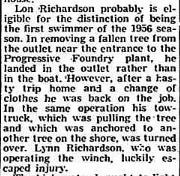This is an image of a newspaper clipping with black text on a white background, framed by thin black lines on either side, with the right side exhibiting a slight gap at the top. The article details an incident involving Lon Richardson, who became an inadvertent swimmer while attempting to remove a fallen tree from an outlet near the entrance to the Progressive Foundry plant. Instead of staying in the boat, he landed in the water. After a quick trip home to change clothes, he returned to the task. Unfortunately, during the same operation, his tow truck, which was anchored to another tree on the shore while pulling the fallen tree, overturned. Lynn Richardson, operating the winch, luckily escaped injury. This snippet suggests Lon is eligible for the distinction of being the first swimmer of the 1956 season due to this mishap.